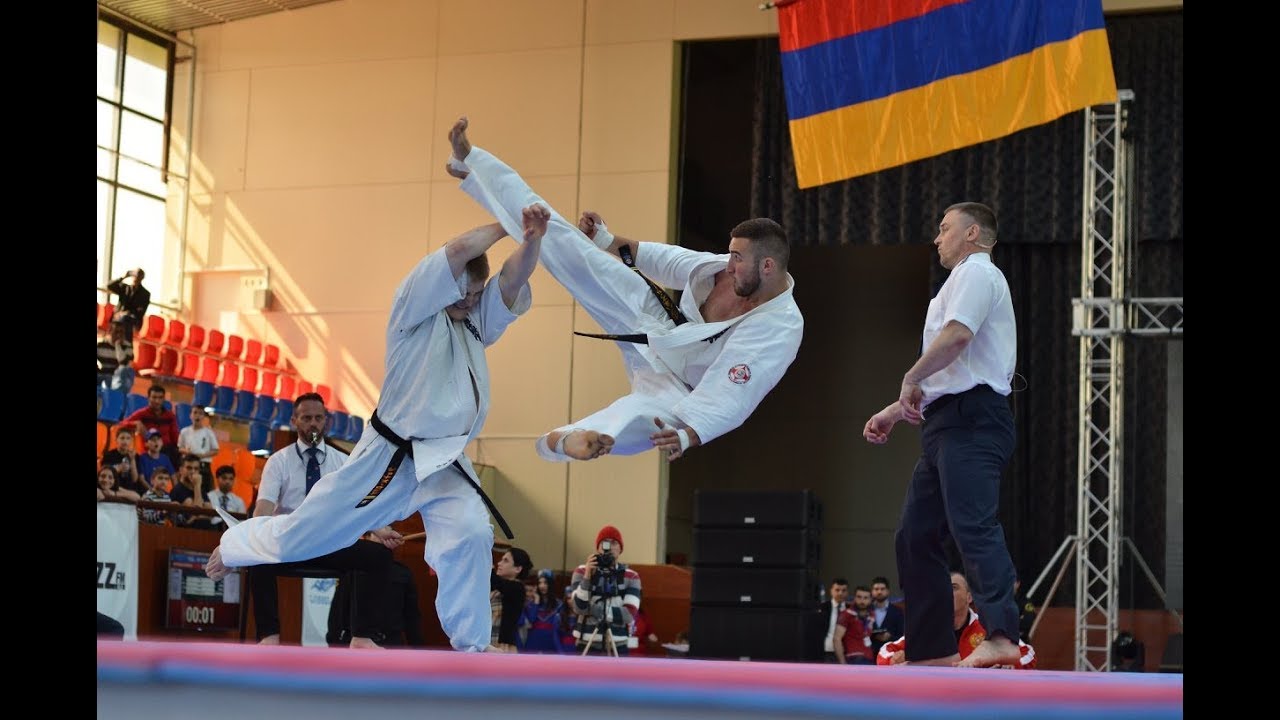This photograph captures an intense martial arts exhibition taking place in a large gymnasium. Center stage, on a matted surface, are two men engaged in a dynamic karate match. The man on the right, barefoot and sporting wrist tape, is airborne in a classic karate pose; his left leg is parallel to the ground while his right leg kicks out powerfully. He has very short hair, a short beard, and is dressed in a kimono-style top. The opponent on the left, with one foot grounded and the other extended behind him, has his arms crossed to intercept the airborne man's outstretched leg. Both seem deeply focused and determined.

Flanking the martial artists are two referees in white short-sleeve shirts with one on the left wielding a whistle. The referee on the right stands attentively, monitoring the match. In the backdrop, a vibrant flag with horizontal stripes of red, blue, and yellow is visible, contributing to the setting's decor. 

Spectators fill the bleachers, bathed in sunlight streaming through the windows, capturing the scene with cameras. Among the audience, there appears to be a table of judges and additional onlookers standing on the gym floor near the stage, all immersed in the excitement of the event.